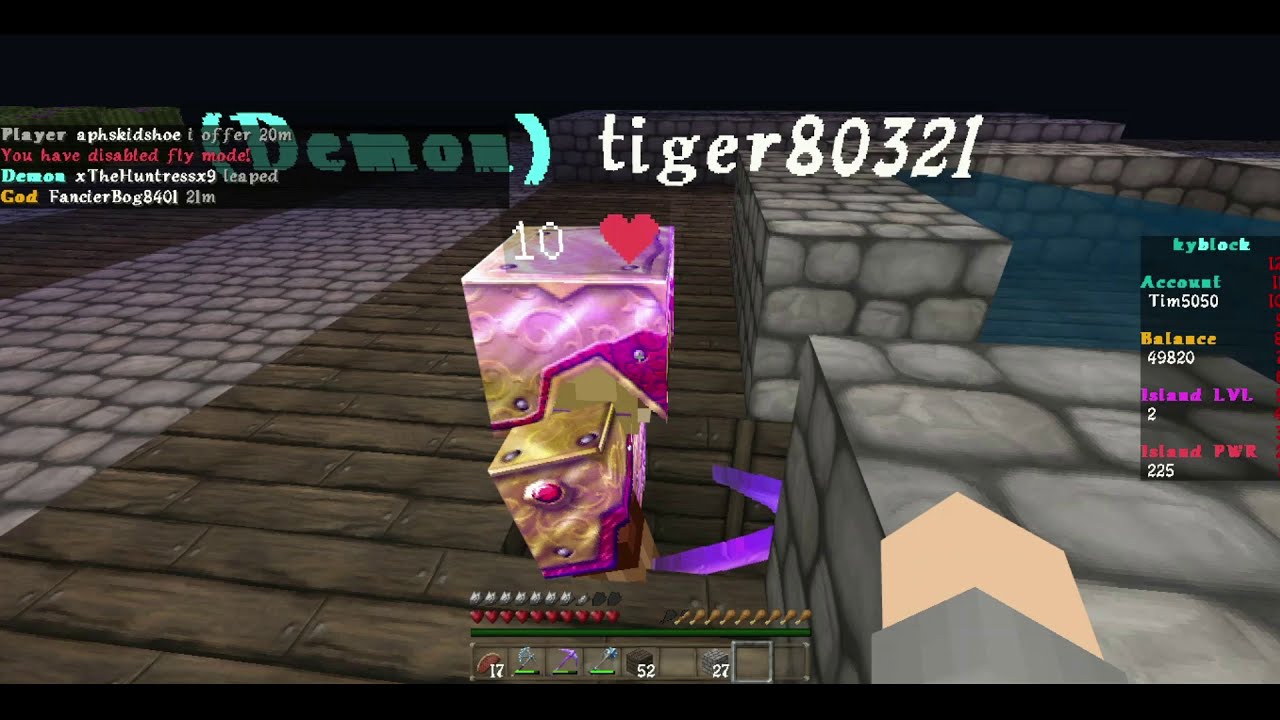The image depicts a video game screen showcasing various player stats and in-game structures. At the top center, in light blue parentheses is the name "Demon," followed by "Tiger80321" in white text. To the right, there is multicolored text: "KY Block" in green, "Tim 5050" in white, a balance of "49820," "Island Level" with the number 2 in purple, and "Island Power" with a score of 225 in red. In the center of the image, the floor is composed of grey brick and brown wooden planks, with symmetrical stone structures on the right forming a short perimeter fence. The middle of the floor features a stack of cubes: purple and pink with a golden cube on top, marked by a white number 10 and a red heart. Along the bottom left, stretches of dark and light purple pavers resemble a roadway, while further detailed text on the right includes "Account," "Balance," "Island," and additional scores. In the top left corner, "Player" is mentioned in white, and the phrase "disabled fly mode" appears in red text. The overall scene is vibrant and detailed, indicating a rich and complex game environment.